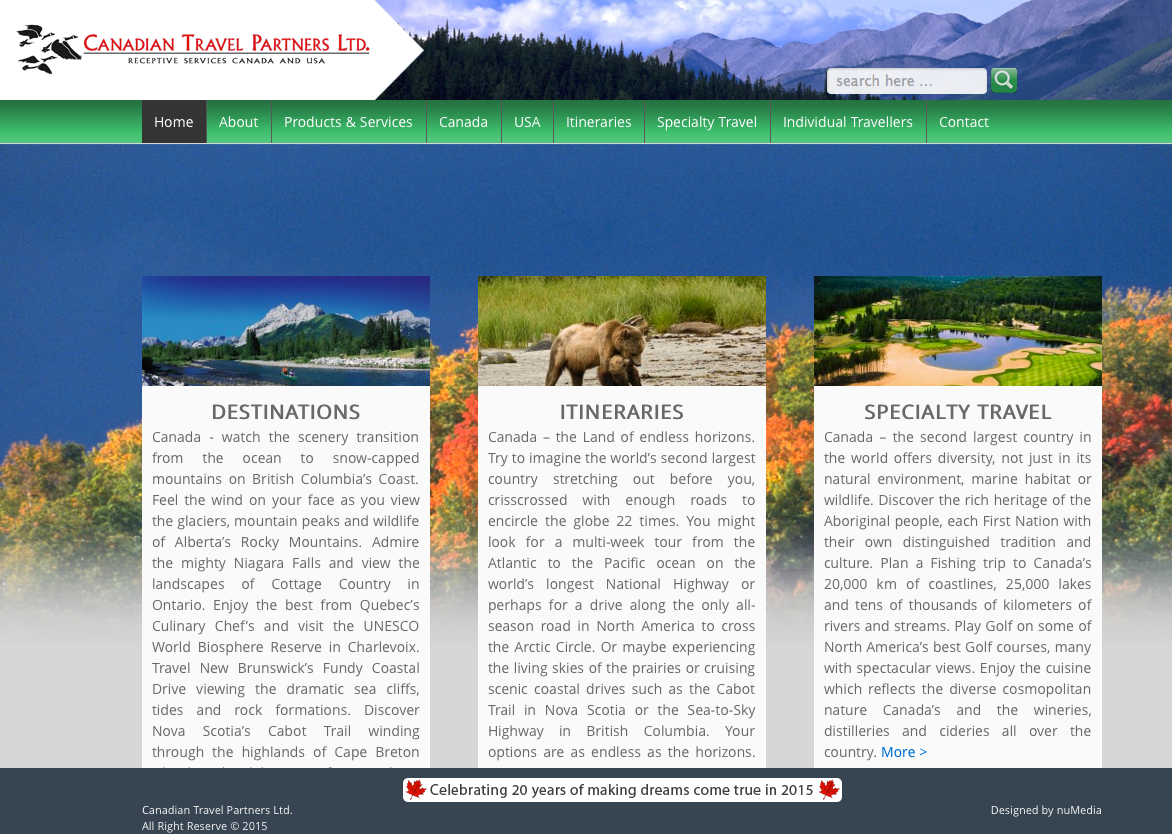A screenshot from the homepage of the Canadian Travel Partners LTD website showcases an organized and visually nostalgic layout. The top banner prominently features an idyllic, forested mountain landscape, evoking the natural beauty of Canada.

Directly below the banner is a navigation bar, offering tabs such as Home, About, Products and Services, Canada, USA, Itineraries, Specialty Travel, Individual Travelers, and Contact, facilitating seamless site exploration.

The current view focuses on the Home tab, which presents three distinct categories: Destinations, Itineraries, and Specialty Travel. Each category is accompanied by a descriptive paragraph. The Destinations section invites visitors to "Watch the scenery transition from the ocean to snow-capped mountains to British Columbia's coast, feel the wind on your face." The Itineraries section encourages travelers to "Imagine the world’s second largest country stretching out before you, a land of endless horizons." Lastly, the Specialty Travel section highlights Canada's vast diversity, not just in its natural environment but also in marine habitats, wildlife, and the rich heritage of the aboriginal people.

At the bottom of the page, a celebratory note mentions, "Celebrating 20 years of making dreams come true in 2015," alongside a 2015 copyright symbol. The bottom-right corner credits the website design to "New Media NU Media," while a convenient search bar is tucked in the top-right corner, rounding off the user-friendly interface.